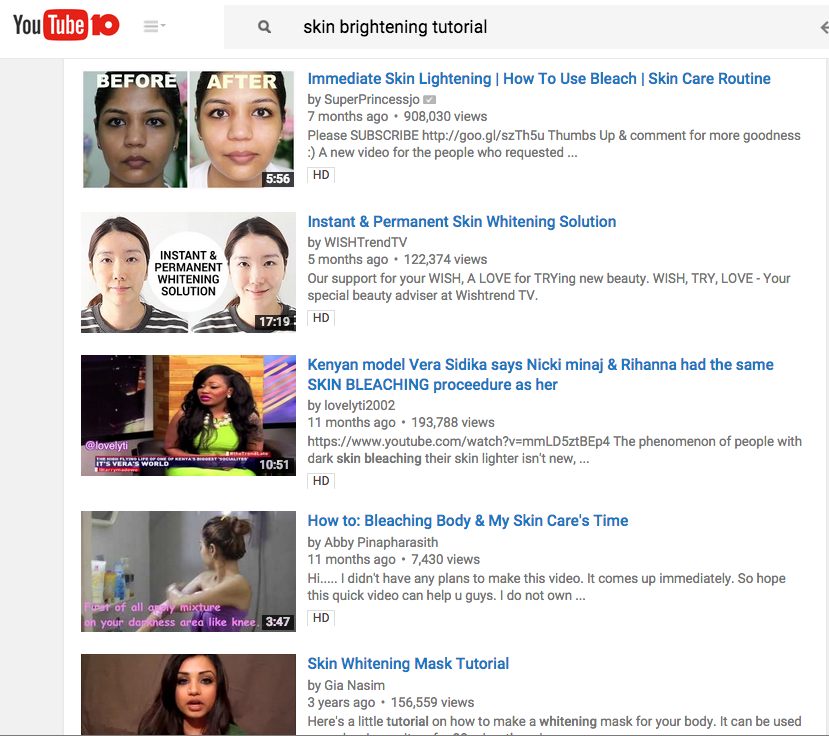The YouTube search results page displays various thumbnails related to skin brightening tutorials. At the top, the YouTube logo is prominently featured with "10" in bold, red lettering. To the left of the search bar, there's an icon with three horizontal lines suggesting additional options. The search query "skin brightening tutorial" is entered in the standard gray search bar, next to a magnifying glass icon representing the search function.

1. **Immediate Skin Lightening Tutorial**  
   - **Thumbnail:** Before-and-after photo of a woman's face, darker on the left panel, lighter on the right.
   - **Video Details:**  
     - Title: "Immediate skin lightening, how to use bleach, skin care routine"  
     - Creator: Super Princess Jo  
     - Duration: 5 minutes and 56 seconds  
     - Views: 908,030  
     - Uploaded: Seven months ago  
     - Additional Info: Subscription link http://goo.gl/scth5u. Encourages viewers to like, comment, and subscribe. Featured in HD.

2. **Instant and Permanent Whitening Solution**  
   - **Thumbnail:** Similar before-and-after comparison with a woman's face.
   - **Video Details:**  
     - Title: "Instant and permanent whitening solution, instant and permanent skin whitening solution"  
     - Creator: Wishtrend TV  
     - Duration: 17 minutes and 19 seconds  
     - Views: 122,374  
     - Uploaded: Five months ago  
     - Additional Info: Promoted by Wishtrend TV as a special beauty advisor channel in HD.

3. **Kenyan Model Veera Siddhika on Skin Bleaching Procedures**  
   - **Thumbnail:** Appears to be a talk show segment.
   - **Video Details:**  
     - Title: "Kenyan model Veera Siddhika: Nicki Minaj and Rihanna used the same skin bleaching procedure as her?"  
     - Creator: Lovely TI 2002  
     - Duration: 10 minutes and 51 seconds  
     - Views: 193,788  
     - Uploaded: Eleven months ago  
     - Additional Info: Link to video includes various character strings. Discussion on the prevalence of skin bleaching.

4. **Bleaching Body and Skin Care Routine**  
   - **Thumbnail:** Woman in a towel facing away from the camera.
   - **Video Details:**  
     - Title: "Bleaching Body and My Skin Care Time"  
     - Creator: Abbey Penifera Siddhika  
     - Duration: 3 minutes and 47 seconds  
     - Views: 7,430  
     - Uploaded: Eleven months ago  
     - Additional Info: The creator did not initially plan to make this video but hopes it helps viewers. Partial text "I do not own…" indicates more information is cut off. Featured in HD.

5. **Skin Lightening Mask Tutorial**  
   - **Thumbnail:** Woman mid-sentence.
   - **Video Details:**  
     - Title: "Skin Lightening Mask Tutorial"  
     - Creator: Gia Nassim  
     - Duration: Not specified  
     - Views: 156,559  
     - Uploaded: Three years ago  
     - Additional Info: Tutorial on creating a lightening mask for the body, though some information is incomplete.

These videos provide various techniques and discussions around skin brightening, showcasing before-and-after comparisons, personal skincare routines, and interviews with public figures on the topic.